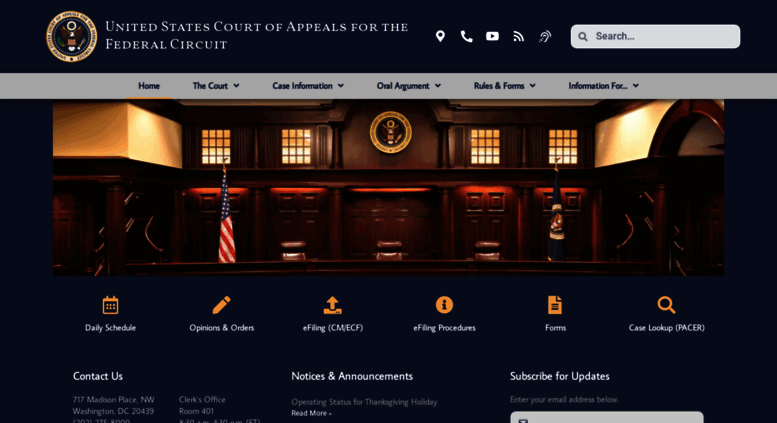In this detailed website screenshot of the United States Court of Appeals for the Federal Circuit, the left section prominently displays the court's name. Adjacent to this, on the right, there's a series of icons: a location icon, a cell phone icon, a YouTube app icon, a Wi-Fi icon, and an icon resembling a sideways hand and wrist. Farther right is a white search bar.

Below these elements are six categories labeled from left to right: Home, The Court, Case Information, Oral Argument, Rules and Forms, and Information For… 

The centerpiece of the image is a photograph of the courthouse, featuring two flags, brown walls, and a brown bench. Beneath this photo, another set of six categories is displayed, with yellow emblems and white text: Daily Schedule, Options and Orders, two unreadable categories, Forms, and Case Lookup.

Further down, the section includes links to Contact Us, Notices and Announcements, and Subscribe for Updates. The entire website background is dark blue, adding a professional and dignified tone to the visual presentation.